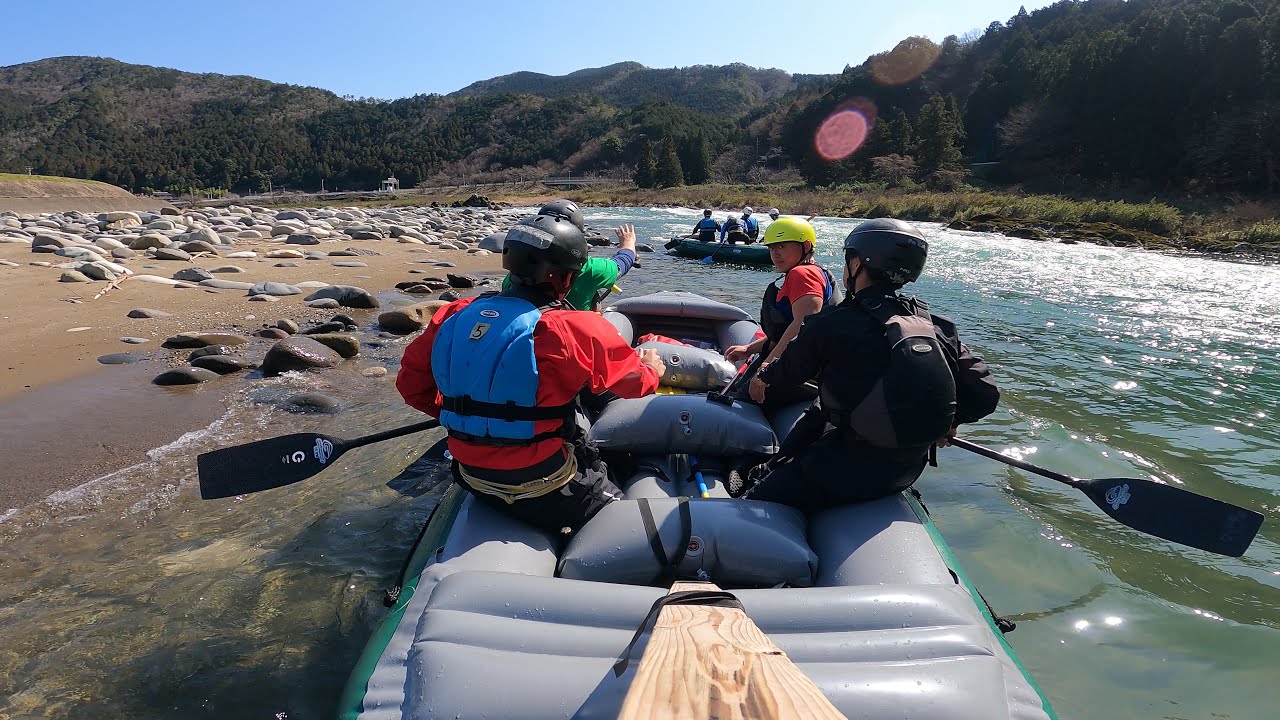In an exhilarating outdoor scene, a group of people is engaged in a rafting adventure on a small river. The main raft, which is gray-green, is captured from the back, showing four people wearing life jackets and helmets, and holding oars. One man on the left is distinct with a blue life jacket and red shirt, while another wears a black life jacket, black shirt, and a backpack. They appear close to a rocky and sandy shoreline on their left while the river stretches out on both sides with a backdrop of majestic tree-covered mountains and a clear blue sky. Another raft can be seen a bit further down the river with its occupants similarly equipped, demonstrating a thrilling yet safe experience amid the serene yet adventurous natural landscape.